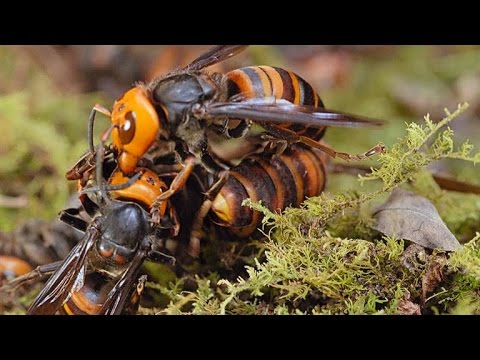In this detailed photograph, two bees appear to be engaged in a mating ritual on a moss-covered ground. The scene features a larger bee at the base and a smaller bee positioned on top. The background, though slightly blurred, showcases a lush carpet of moss. The bees possess distinctive coloration: they have solid orange heads, with the bee on top displaying a prominent, round, brown eye. Their bodies are predominantly black, transitioning into alternating black or dark brown and orange stripes along their abdomens. The smaller bee beneath has notably larger legs and a head with less orange coloration compared to its counterpart. The intricate details and the unique color patterns of these bees provide a captivating look at this moment in nature.